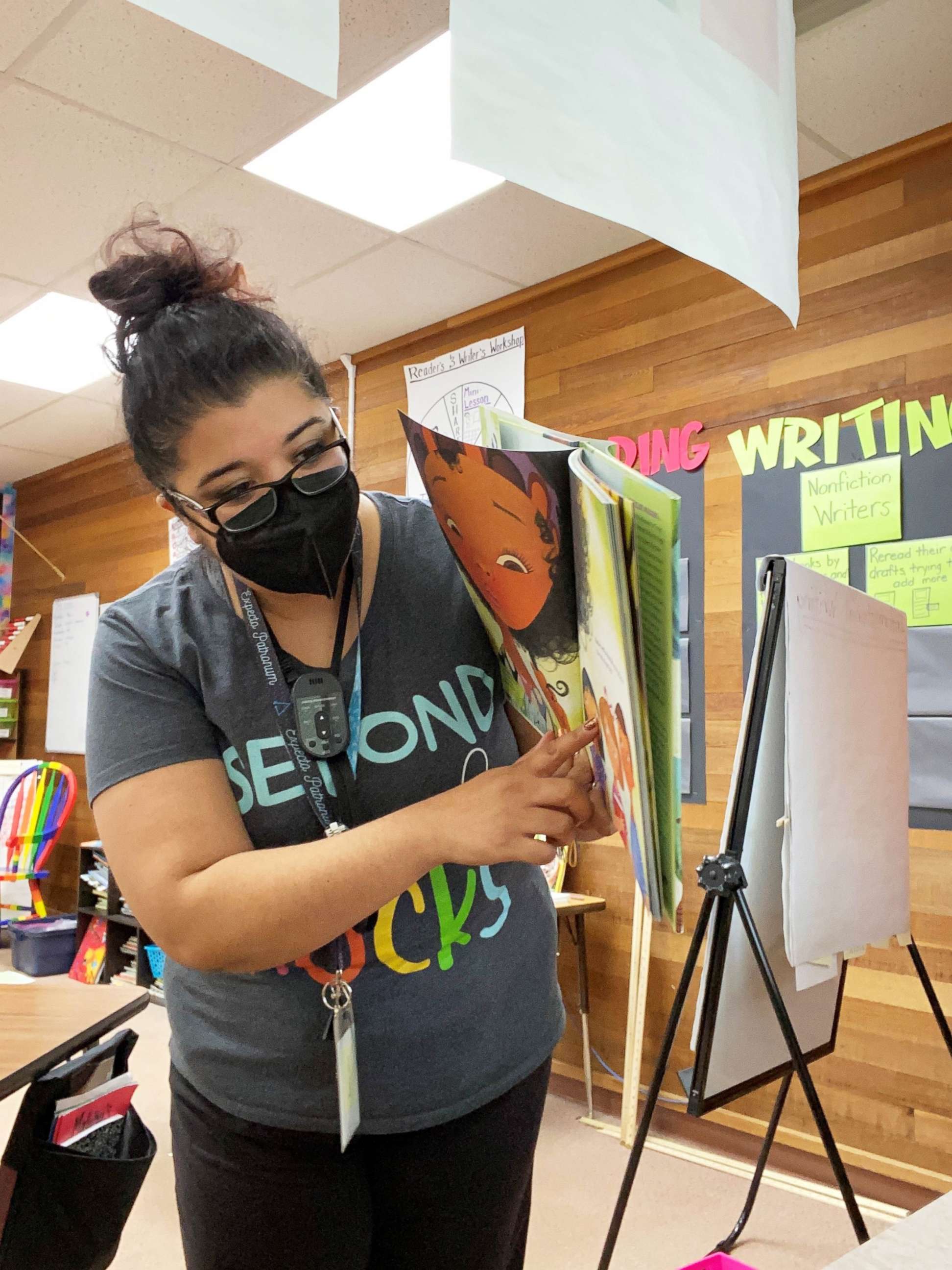The image depicts a slightly overweight Latina woman with slightly tan, light brown skin and curly brown hair styled in a small bun on top of her head. She is standing in what appears to be a classroom environment, indicated by the wooden tabletop and chair with a backpack on it to her left, an easel with flipped-over paper to her right, and multicolored posters and items on the wooden slat wall behind her. The wall features various educational materials, including something labeled "writing," and there are items hanging from the ceiling as well. The room is illuminated by fluorescent lights from a white ceiling.

The woman is holding a children's book in one hand and pointing to a character in the book with the other, as if she is exhibiting it to a class of children, though no children are visible in the frame. She is wearing black plastic eyeglasses, a black face mask, a gray t-shirt with some writing on it, black pants, and a lanyard, which possibly holds work-related items. She also appears to be wearing a wristwatch. In the far background, there is a rainbow-colored chair, and the visible carpet is beige. The overall scene suggests she is engaging with students in a teaching capacity.